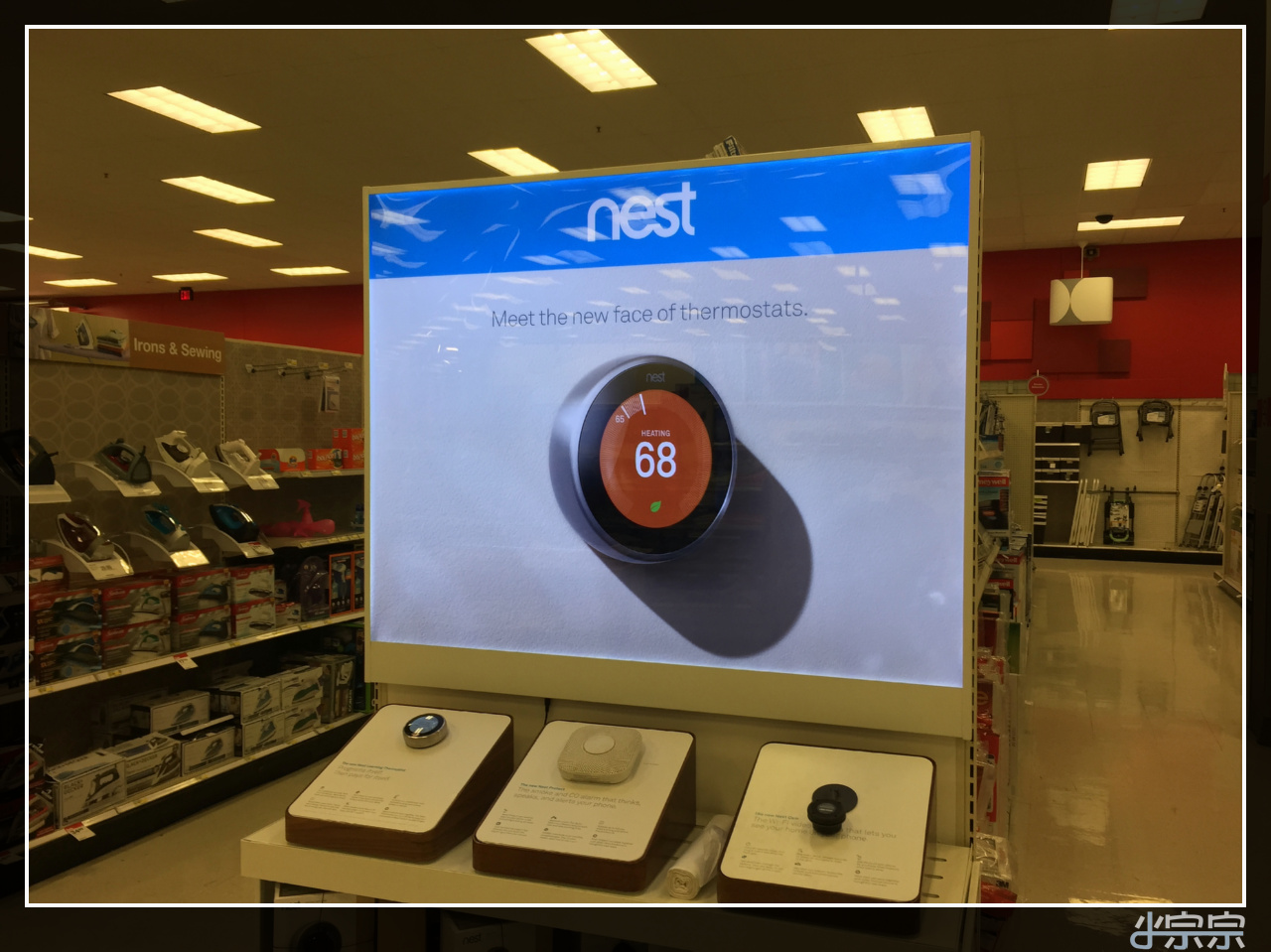In this photograph, taken in what appears to be an electronic or department store, the background features a ceiling with multiple rectangular lights, all of them turned on, casting a bright, uniform illumination throughout the space. To the very right, an empty corridor extends into the distance, with shelves unseen but suggesting a continuation of the store's layout. To the left, another corridor comes into view, showcasing a display of electronic equipment, possibly telephones neatly lined up on the shelves.

Dominating the center of the frame is a prominent sign with a blue stripe at the top reading "Nest," followed by the phrase "meet the new face of thermostats." The centerpiece of this sign is a round, black thermostat with an eye-catching red face. The thermostat displays the temperature "68" in bold white numerals, accompanied by a small green dot below the number, indicating its active status. The thermostat is presented with an exaggerated shadow, adding a sense of depth to the image.

Beneath the sign, there is a display featuring three distinct models of the same Nest thermostat, each representing a different variation of this innovative device. The meticulous arrangement and clear signage direct the viewer's attention, emphasizing the advanced features and sleek design of the Nest thermostats.